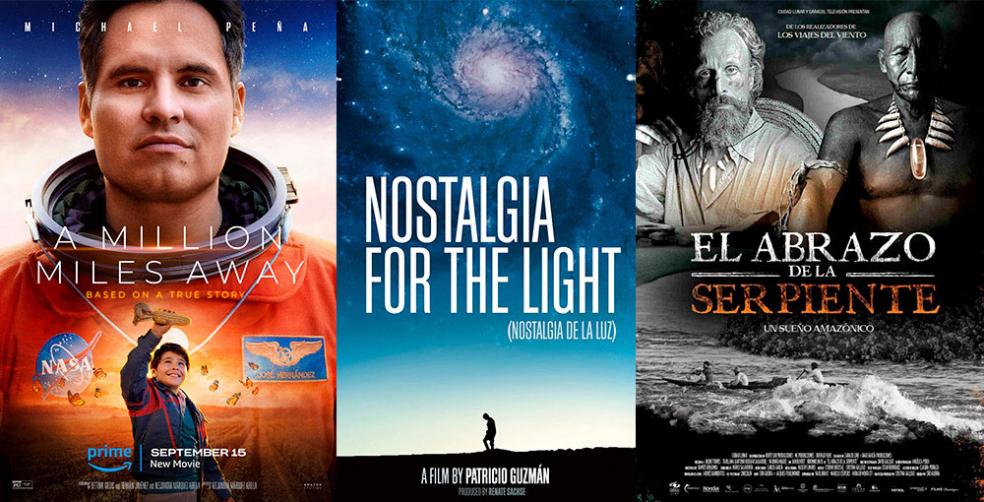The image is a rectangular advertisement, about six inches wide and two inches tall, divided into three sections for different movies. 

The left section is a poster for "A Million Miles Away," featuring a serene man in a spacesuit without a helmet. The top of the poster highlights actor Michael Peña and the film's title, along with the tagline "Based on a true story." Below, a young boy joyfully flies a wooden rocket ship over his head, with the NASA logo to his left. The man's spacesuit also reveals the name "Hernandez." The film is advertised for release on Amazon Prime on September 15th.

The middle section showcases "Nostalgia for the Light" (Nostalgia de la Luz), a film by Patricio Guzman. The background displays a cosmic vortex, and a silhouette of a man walks dejectedly along a path at the bottom of the poster. The title is prominently placed in white print along with the film's bilingual title.

The right section advertises "El Abrazo de la Serpiente" (Embrace of the Serpent), subtitled "Un Sueño Amazónico." The top half of this poster features two men: one of Caucasian descent wearing a white colonial shirt and a spiked necklace, and the other of apparent Native American descent with a bushy beard and a similar necklace, enhanced with a prominent turquoise gem. Below these figures, people navigate a canoe through white-water rapids.

Together, the three sections highlight evocative movie imagery and thematic elements, ranging from space exploration and cosmic reflection to cultural encounters and adventures on the Amazon River.